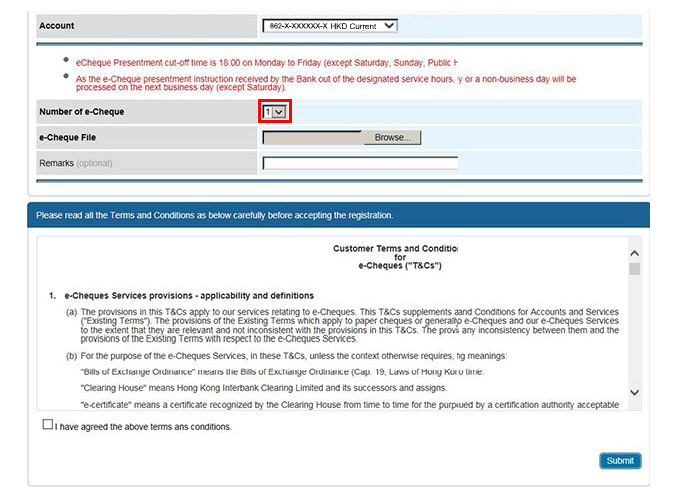This is a detailed screenshot from a website, primarily featuring a financial form for E-check submission. The layout consists of predominantly black text on a white background, with a gray bar at the top labeled "Count." This bar contains a fillable field for users to enter a number, although it's currently filled in with placeholder text "XXX" that isn’t completed properly.

Beneath this section, in red text, the instructions read "E-check, Presentation, Presentment, Cut off time is 1800 on Monday to Friday, except Saturday, Sunday." Further down, it states that "E-check presentment instructions received by the bank outside designated service hours or on a non-business day will be processed the next business day, excluding Saturday." 

There is a small box labeled "Number of E-checks" which contains the number "1." This displays a red rim superimposed around it. Below, there is an area labeled "E-check file" with an option to browse and upload a file. Additionally, there is an "Optional Remarks" field.

A blue band with white text reads, "Please read terms and conditions below carefully before accepting the registration. Customer terms and conditions for E-checks are written below." Following this, it details the "E-check Service Provision, Applicability and Definitions," presented in sections labeled A and B. The text in these sections is particularly small and not well-rendered, making it difficult to read.

At the bottom of the form, there is a checkbox for users to agree to the terms and conditions, labeled "I agree to both terms and conditions," which remains unchecked. Adjacent to this is a blue submit button.

Notably, there's a suspicious element – an error in the language used in the red-highlighted section near the E-check instructions. The phrase uses “A-N-S” instead of “A-N-D,” which raises concerns about the legitimacy of this website, especially given its financial context. This language discrepancy suggests the potential that this could be a scam website.